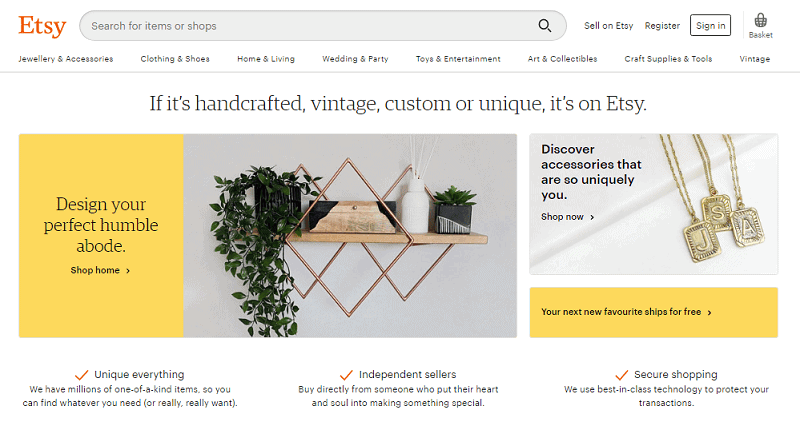This screenshot captures the Etsy homepage, showcasing various features and highlights. At the top, there is a search bar labeled "Etsy: Search for items or shops," accompanied by options to "Sell on Etsy" and "Sign in." Below this, the different shopping categories are neatly listed: Jewelry & Accessories, Clothing & Shoes, Home & Living, Wedding & Party, Toys & Entertainment, Art & Collectibles, Craft Supplies & Tools, and Vintage.

A tagline emphasizes Etsy’s unique offerings: "If it's handcrafted, vintage, custom, or unique, it's on Etsy." Prominently featured is a yellow box with the text, "Design your perfect, humble abode. Shop Home," next to an image of a floating shell-like shelf adorned with a plant, a small chest, a succulent, and incense.

Adjacent to this, another section invites users to "Discover accessories that are so uniquely you," featuring three necklaces with initials "J," "S," and "A," encouraging users to "Shop now." Below the necklaces, another yellow box states, "Your next new favorite ships for free."

At the bottom, Etsy reassures shoppers with statements about the platform's uniqueness and security: "Unique everything: We have millions of one-of-a-kind items so you can find whatever you need or really, really want." Additionally, it highlights the personal touch of shopping on Etsy: "Unique independent sellers: Buy directly from someone who put their heart and soul into making something special." Lastly, it affirms the safety of transactions with, "Secure shopping: We use best-in-class technology to protect your transactions."